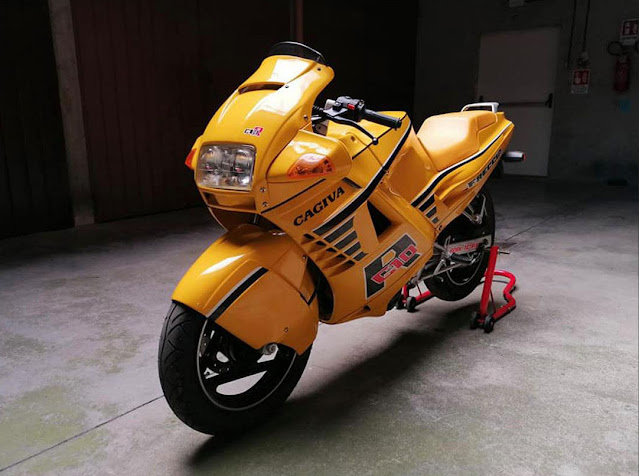This photograph depicts a striking, vintage sporty motorcycle from the 80s style, predominantly painted in yellow with minor black stripes. The body, seat, and front fascia, including the headlight cover and side mirrors with integrated turn signals, all share the vibrant yellow hue. The smooth front wheel cover extends halfway down the wheel. The motorcycle's dark elements include the handlebars, tires, and writing on the side, which reads "CAGIVA" in black text. Additionally, there are large, bold letters near the engine area: a black 'R' with a white outline and 'C10' red letters with a white outline, likely indicating the model type. The motorcycle stands on a concrete floor in a garage-like setting, with its back wheel elevated by a red stand that features wheels for mobility. Behind the motorcycle, a closed white door is visible, further emphasizing the abandoned ambiance.